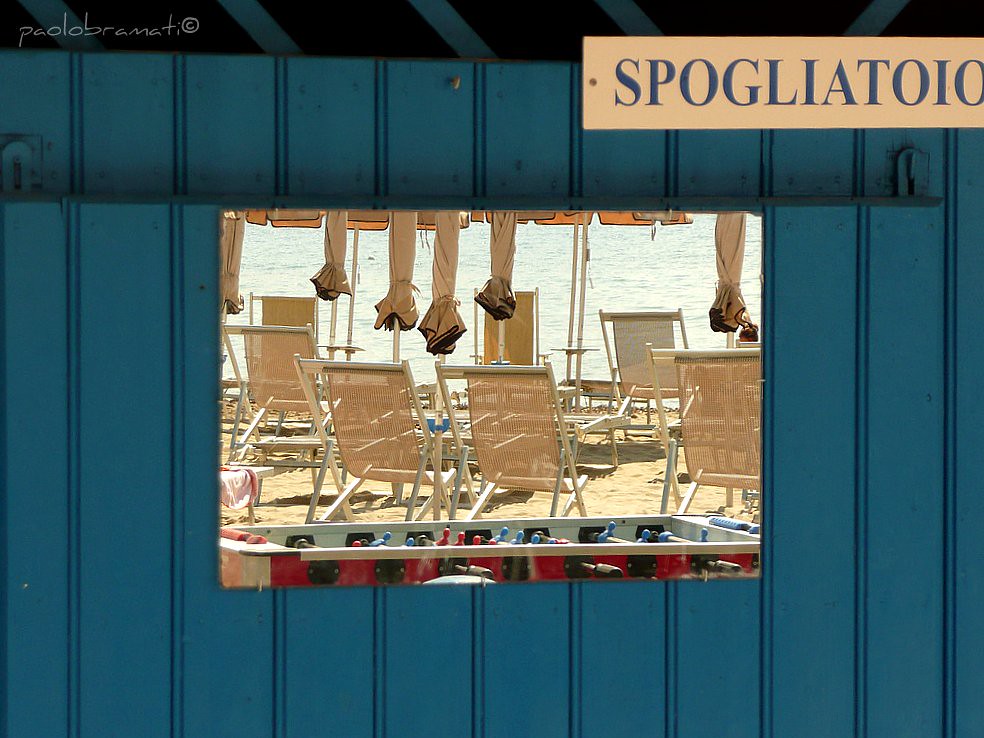The photograph depicts a wall composed of dark teal to marine blue wooden panels, which might belong to a shed or similar structure. Mounted on the wall is a canvas painting of a beach scene featuring several beige foldable lounge chairs and tan-colored, tightly wound umbrellas. The background of the painting shows water with light greenish ripples, indicating a sunny day with shadows cast on the sand. In the foreground, there's a vibrant red foosball table with black handles and blue and red players. The photograph bears a watermark in the top left corner that reads "Paolo Bramati."